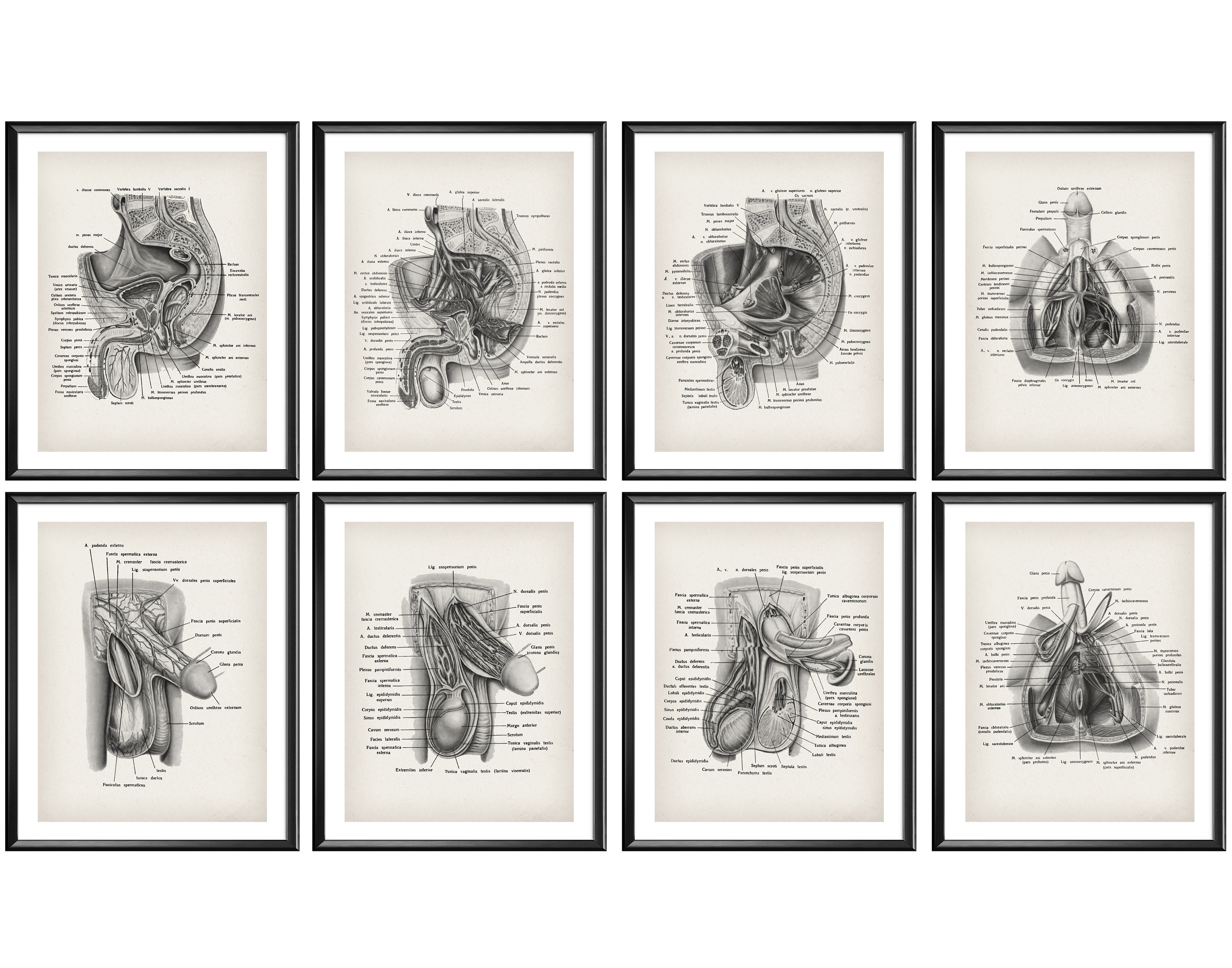This image features a collection of eight framed anatomical illustrations, specifically focused on the male genitalia. Each illustration, drawn in black on a tan background, meticulously labels various parts of the male reproductive system with lines and text. The frames have a distinctive design, featuring a white border immediately around each illustration, followed by a surrounding black border, all set against a plain white background. The series details the internal and external anatomy of the male genitals, with particular emphasis on the penis and its associated structures. On the bottom row, several images depict an erect penis from different angles, including side views and a top-down perspective. Due to the small print, the specific glands and ducts are difficult to read, but the overall artistic and scientific effort to showcase the male reproductive system is evident in this detailed collection.